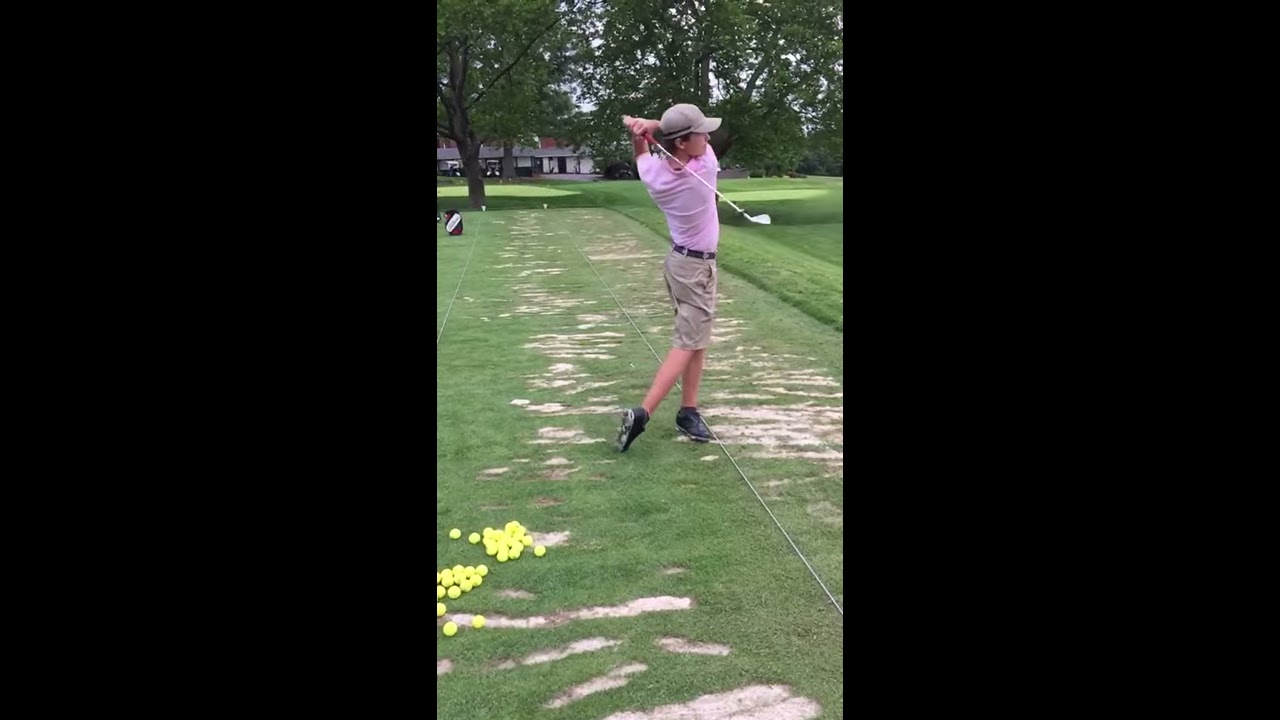In this detailed image, a man is captured mid-swing at a golf driving range. The scene is set on a green, though notably patchy, grassy lawn scattered with numerous yellow golf balls. The man is wearing a light purple (polo) shirt paired with khaki shorts, black shoes, and a gray hat. He stands with a golf club positioned over his left shoulder, suggesting he has just completed a swing. He is looking to the right side of the image, presumably to track the ball's flight. The backdrop features trees and a building where several vehicles are parked, indicating it’s a public or club facility. The overall scene is slightly marred by the patchy grass with visible dirt areas, detracting from the pristine conditions typically expected of a golf setting. The photograph, taken in portrait orientation, is bordered by vertical black strips on both the left and right sides, which frame the central subject.